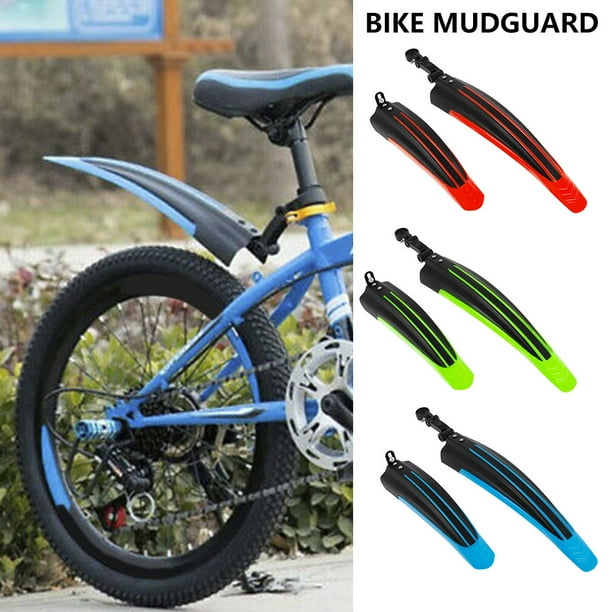In this advertisement for bike mudguards, the top right corner in bold black lettering reads "Bike Mudguard." The ad showcases three sets of mudguards in various colors: black with red tips, black with neon green tips, and black with light blue tips. On the left half of the image, there's a detailed outdoor photo of the back half of a bike. This part of the image shows a black seat mounted on a post, with a black mudguard attached directly underneath, extending over the rear tire to prevent mud from splashing onto the rider’s back. The bike appears to be stable on a kickstand, with a wooden sign and shrubs in the background, indicating it was taken during the daytime. Additionally, the rear tire's spokes, chain, and center crank wheel are clearly visible. The right half of the ad arranges the three sets of mudguards in vertical rows: the top row features black mudguards with red tips, the middle row displays black mudguards with neon green tips, and the bottom row shows black mudguards with light blue tips. The ad effectively combines both detailed product images and the practical application of the mudguard on a bike.